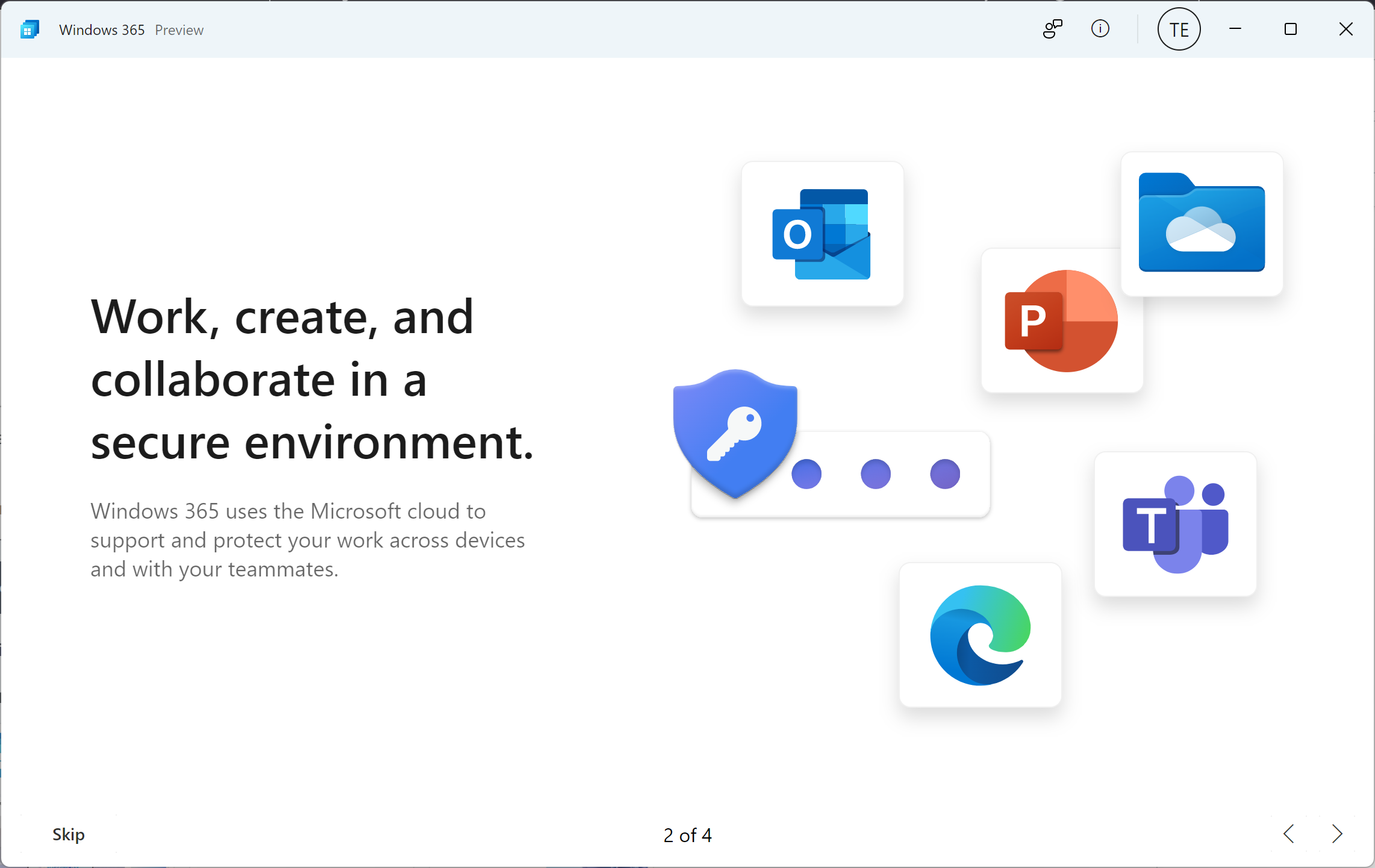This is a detailed screenshot of a Windows 365 preview window. At the top of the window, there is a very pale blue taskbar featuring a stacked Windows icon, composed of four blue squares, indicating the Windows logo. To the right of the logo, there's a series of icons: a line drawing of a person with a speech bubble, an eye in a circle, and the initials "TE" in a circle, likely representing the account owner's initials. Additionally, the taskbar includes standard window controls: minimize (a dash), maximize (a rounded square), and close (an X).

Below the taskbar, on a white background, black text reads, "Work, create and collaborate in a secure environment." In gray font beneath that, it explains, "Windows 365 uses the Microsoft Cloud to support and protect your work across devices and with your teammates."

Further down, several program icons are displayed:

1. **Outlook**: A blue letter emerging from a blue envelope with a blue "O" in a rounded square overlay.
2. **PowerPoint**: An orange-red rounded square with a white "P" in front of an orange-red pie chart.
3. **Cloud Files**: A blue folder with a white cloud accented by light blue highlights, alongside a purple shield with a key and ellipses.
4. **Microsoft Teams**: Two figures, one light purple and one dark purple, next to a rounded square containing a white "T."
5. **Microsoft Edge**: A logo resembling a cresting wave with a blue base that gradients to green at the top.

At the bottom of the screenshot, navigation options are visible: an option to skip, an indicator showing this is page 2 of 4, and forward and backward arrows.